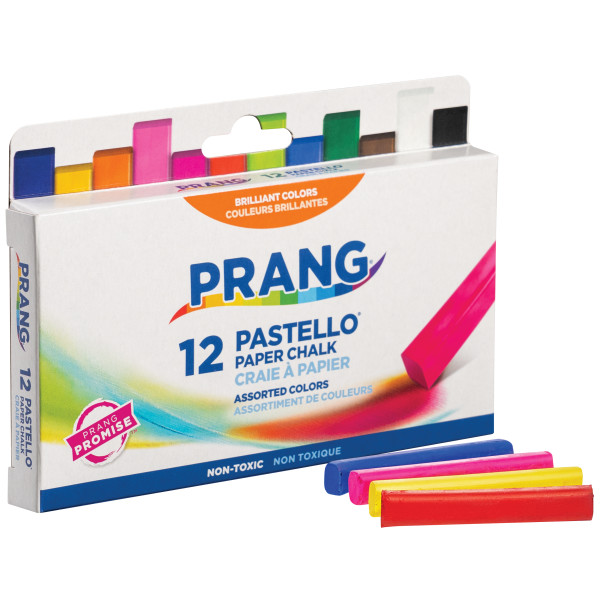The image showcases a neatly arranged product of Prang’s 12 Pastello Paper Chalk sticks set against a white background. The packaging is a long, narrow, white rectangular box adorned with simple blue lettering and an orange swoosh above the brand name "Prang." The box features both English and French text, indicating it is a bilingual product. Prominently displayed on the front of the package, the words "12 Pastello Paper Chalk Assorted Colors" are visible, accompanied by the French equivalent "12 Pastello, Papillon de Couleur." The front also depicts a lively illustration of chalk making a colorful mark. At the top of the packaging, one can glimpse several colors of chalk protruding, including blues, yellows, greens, white, and black. To the left side, the “Prang Promise” emphasizes the brand’s commitment to quality. In front of the box, four individual chalk sticks are laid out: one blue, one pink, one yellow, and one dark red. This detailed product image highlights the vibrant and assorted colors included within the set, making it a compelling advertisement for Prang's non-toxic Pastello Paper Chalk.